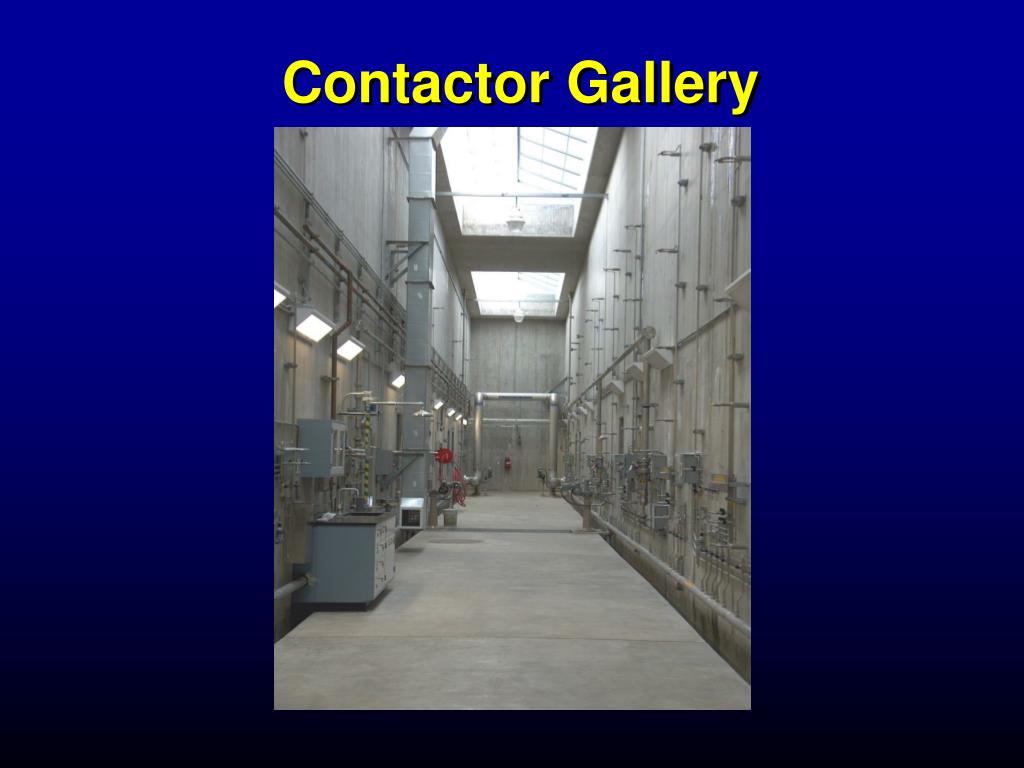The image is part of a slideshow set against a blue background, featuring a central photograph of an industrial factory or power plant interior. The top of the image bears the title "Contractor Gallery" in prominent yellow font. The factory space depicted is a long, narrow corridor with a high, glass-ceiling that allows natural light to flood in. This area has concrete floors and is dominated by numerous silver-colored metal pipes running along both walls. These walls also feature multiple gauges, switches, plugs, and electrical components. Among the varied industrial elements present, a notable red pipe is positioned further down the space. The overall aesthetic appears futuristic yet grounded in reality, painted with an industrial gray palette. The meticulous arrangement of various factory apparatuses and the cleanliness of the scene contribute to an impression of precision and functionality.